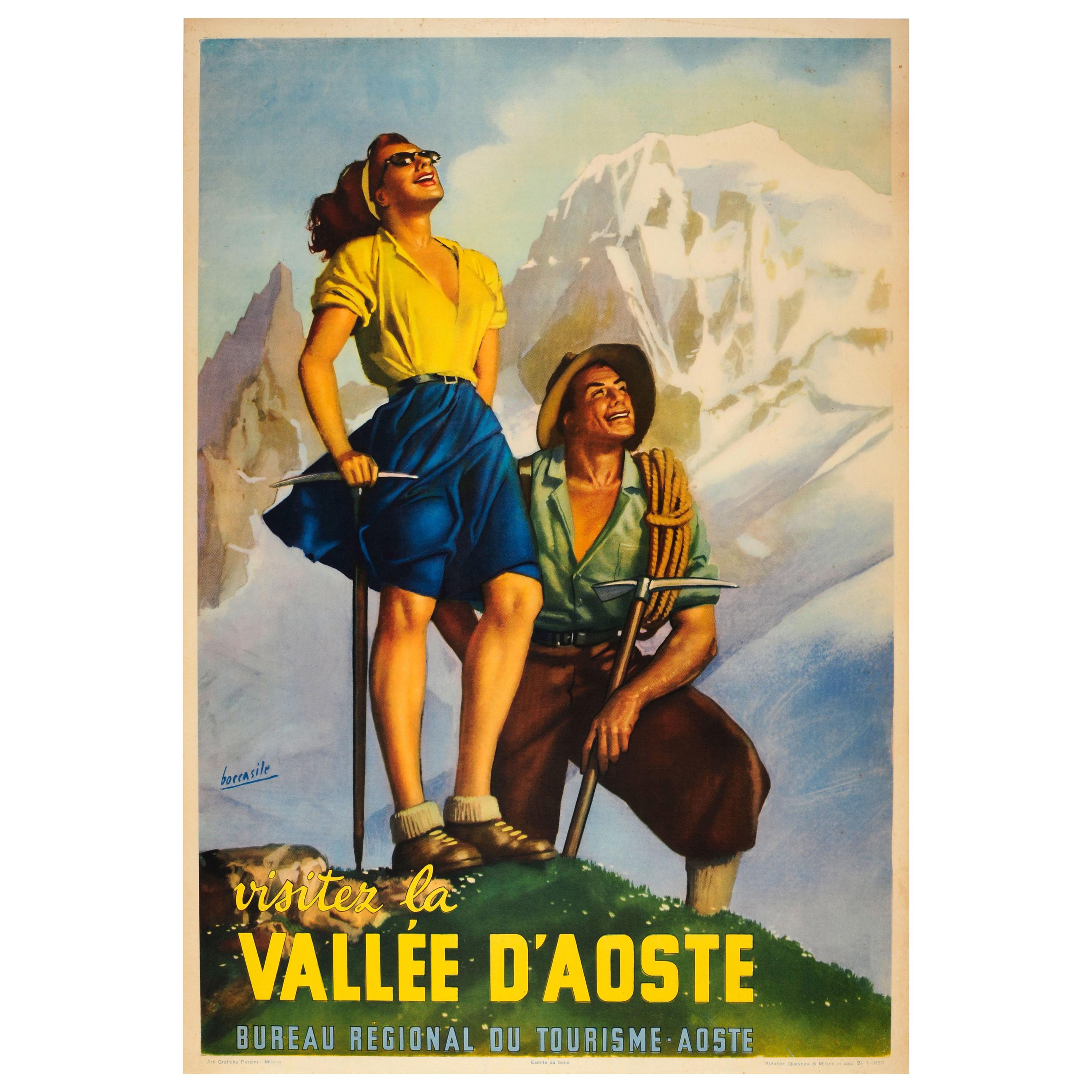The image is a vintage-style advertisement for a tourist magazine or visitor's guide, likely from the early 50s, with a narrow, light brown border. Set against a backdrop of snow-capped mountains and a blue sky, it features two people on a green and rocky knoll. On the right side of the knoll, there is green grass, while the left side transitions to brown rocks. 

The woman, who has light skin, long blonde hair pulled back with a yellow band, is dressed in a blue skirt, a short-sleeved white blouse, and sunglasses. She stands upright, using a pickaxe like a walking stick, her face tilted upwards as if enjoying the sunlight. The man, also light-skinned and dressed in short gaucho pants, a buttoned-up blue shirt, and a broad-rimmed hat, is kneeling beside her. He has a rope draped over his left shoulder and holds a pickaxe.

In bold yellow letters across the image, it reads "Visit La Vallée d'Aoste." Below this, in blue print, is "Bureau Régional du Tourisme." The background suggests an alpine setting, emphasizing the juxtaposition of their summer attire against the snow-covered peaks.